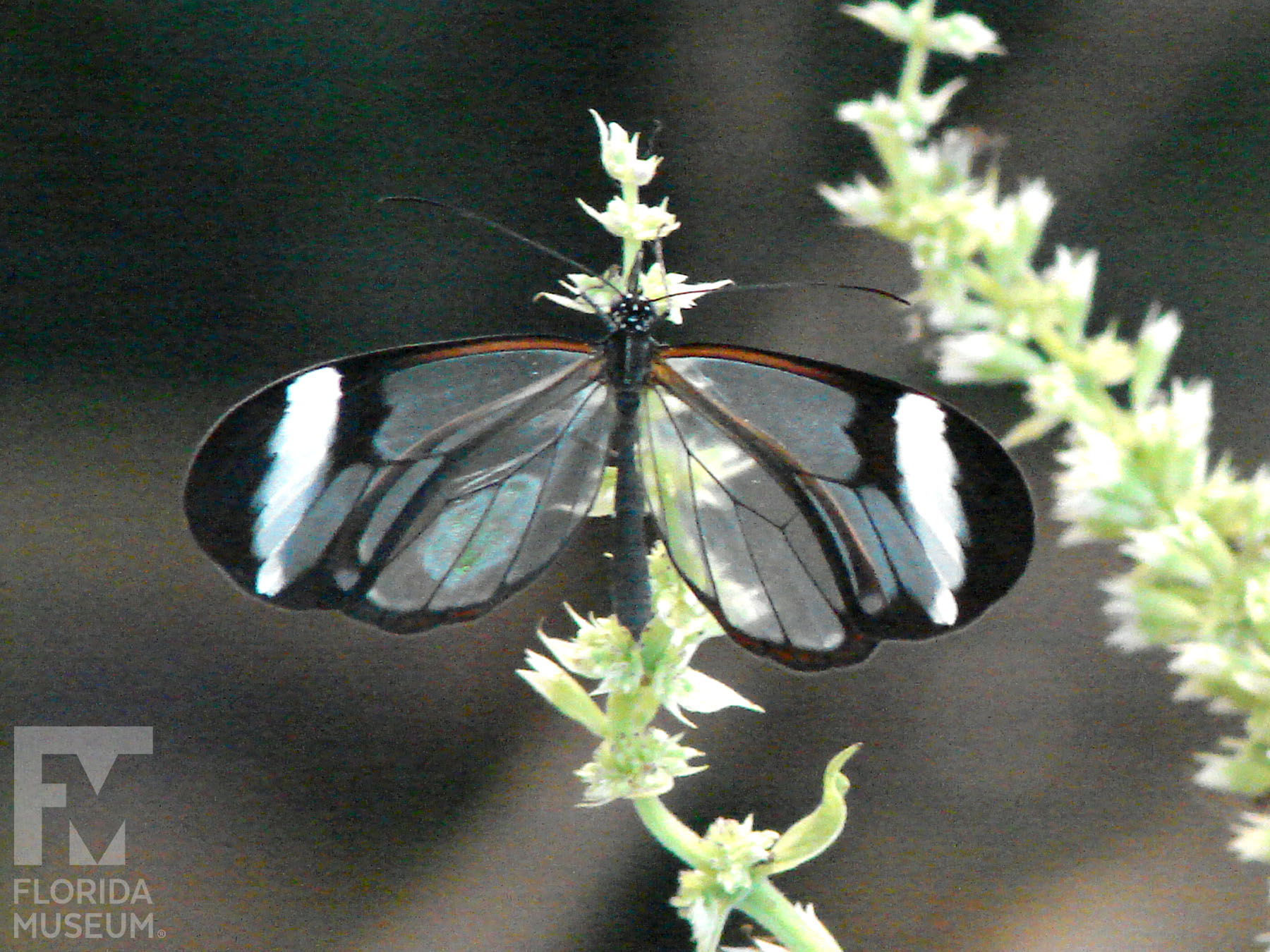This detailed photograph from the Florida Museum captures a distinctive butterfly perched on a green plant with clusters of small, white-petaled flowers. The butterfly's wings are a striking feature, being mostly transparent with a slight iridescence covering about two-thirds of them. The edges of its wings are tipped with black, each featuring a vertical white stripe towards the end. It has long, slender black antennae extending from its head. The scene appears to be bathed in natural daylight, likely captured during the early morning or noon as the sunlight seems to shine directly above the butterfly. This precise moment is accentuated by the blurred background that focuses the viewer's attention on both the butterfly and the plant it rests on. The image is affirmed to be from the Florida Museum, with the institution’s logo and name - a stylized white square with an "FM" within it - prominently displayed in the bottom left corner along with the accompanying copyright symbol.